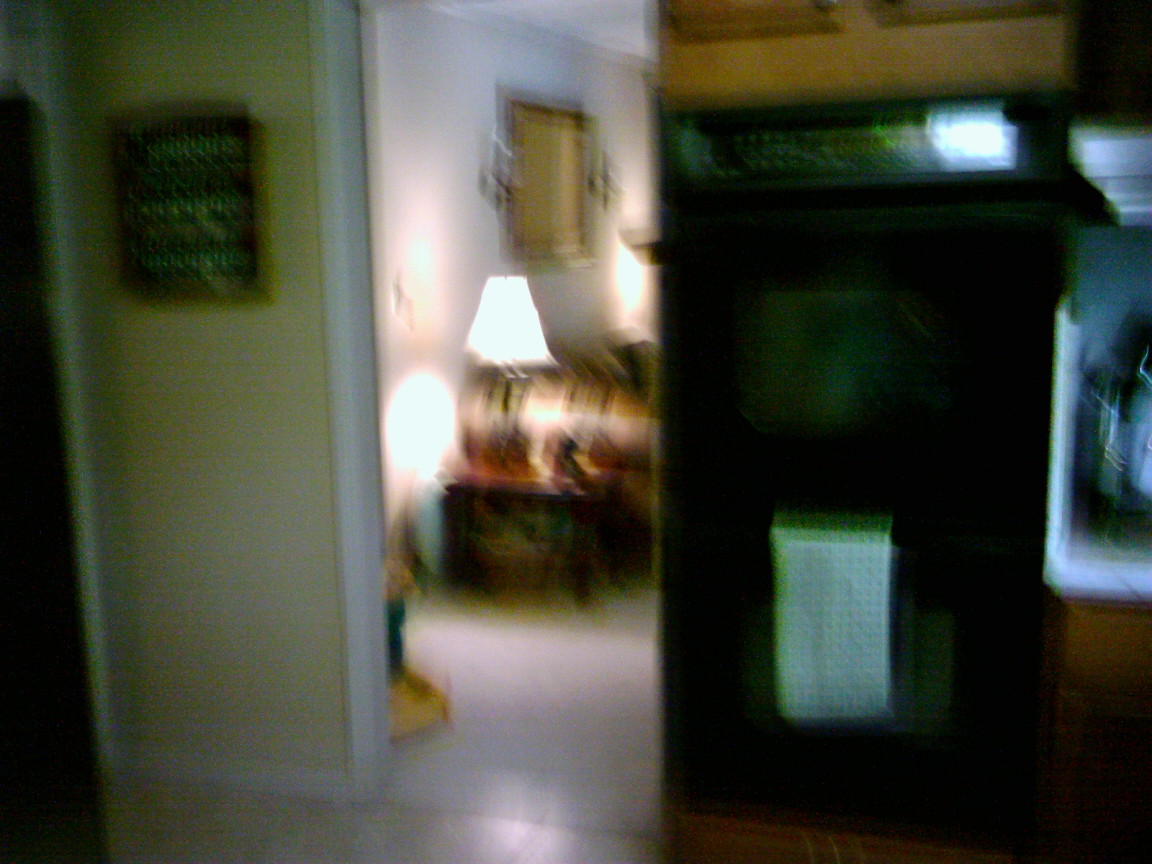This extremely blurry, horizontally aligned indoor photograph captures a view from the kitchen, looking through a doorway into a living room. The kitchen has yellow walls with a white border and baseboard, wooden cabinets above, and a white countertop cluttered with dishes. A black stove beneath the cabinets has a towel draped over the handle. To the right of the stove stands a potentially black refrigerator. 

The doorway opens into a well-lit living room. A large white-framed mirror hangs on the wall behind a striped brown couch. Beside the couch is a black or wooden coffee table with a lit lamp featuring a white lampshade. The lamp illuminates a picture hanging above the couch, further detailing the cozy interior.